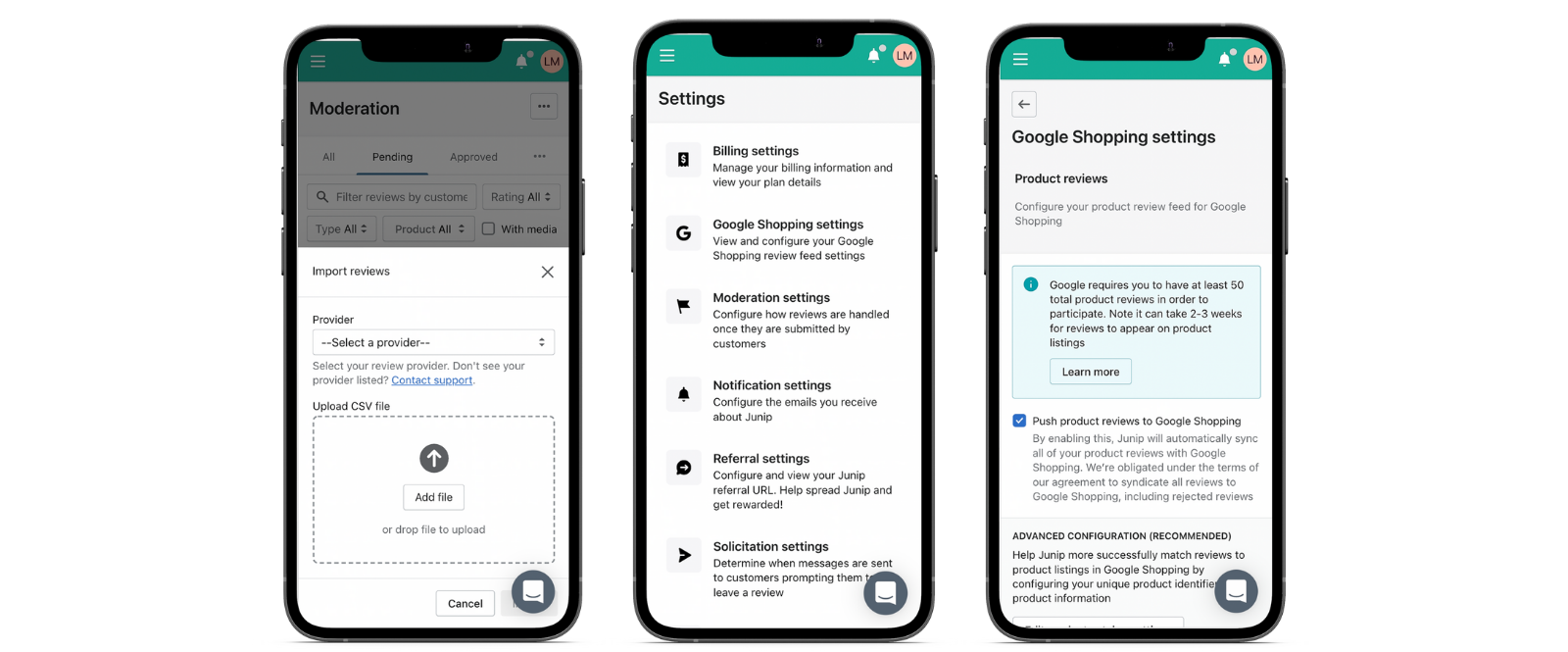In the image, three smartphones are displayed, each showcasing different screens and interfaces:

1. The first smartphone features a green banner at the top with a small shopping cart icon. Below this, a purple box labeled "Moderation" contains text that is underlined in blue. The remainder of the screen is white, displaying the options "Import," "Print," and a square icon with an upward arrow.

2. The second smartphone presents a teal-colored bar at the top. The screen, predominantly white, displays "Settings" along with varied options and categories under "Google Shopping Settings."

3. The third smartphone also has a teal top banner stating "Google Shopping Settings" alongside a section titled "Perfect Movies," marked by a small green box and circle next to it. Below, there is another green box accompanied by a check mark and a paragraph. The bottom portion of the screen contains text written in purple.

The detailed elements on each screen suggest they are related to differing aspects of app functionality and settings for e-commerce or content management.